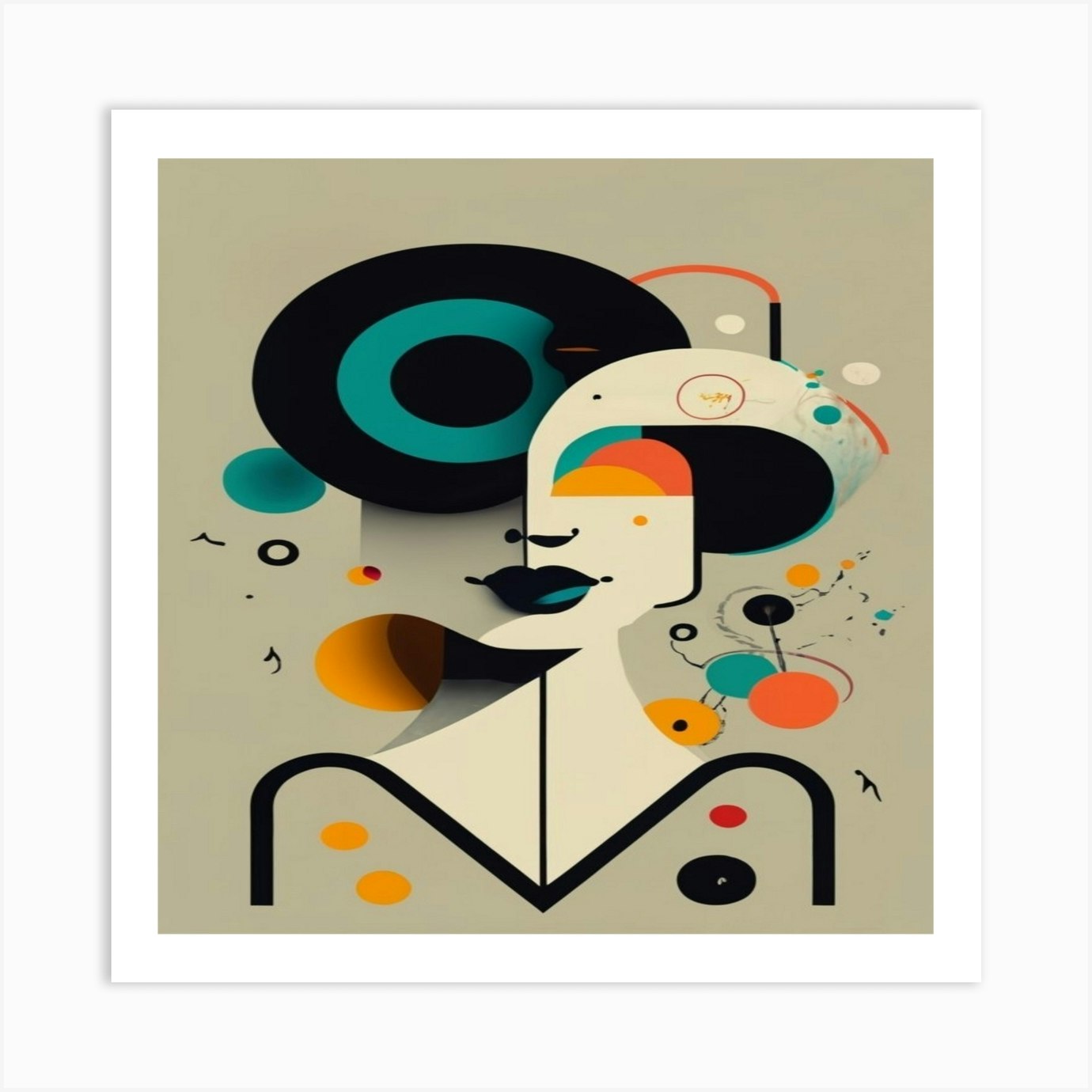The image shows a stylized, abstract painting of a woman set against a beige background, framed by a white border. The painting emphasizes exaggerated shapes and features in a whimsical style. The woman's lips are defined by teal and black, but her hair and eyes are either indistinguishable or creatively depicted, with one eye represented as a record. Her figure is suggested in broad strokes, adorned with various colors. Surrounding her are vibrant, randomly placed circles and splotches in hues of teal, black, pink, orange, and yellow, contributing to the funky, dynamic feel of the artwork. Notable features include a group of concentric circles in the upper left and an orange line pointing downwards. The painting's playful details and use of color create a lively, captivating composition.